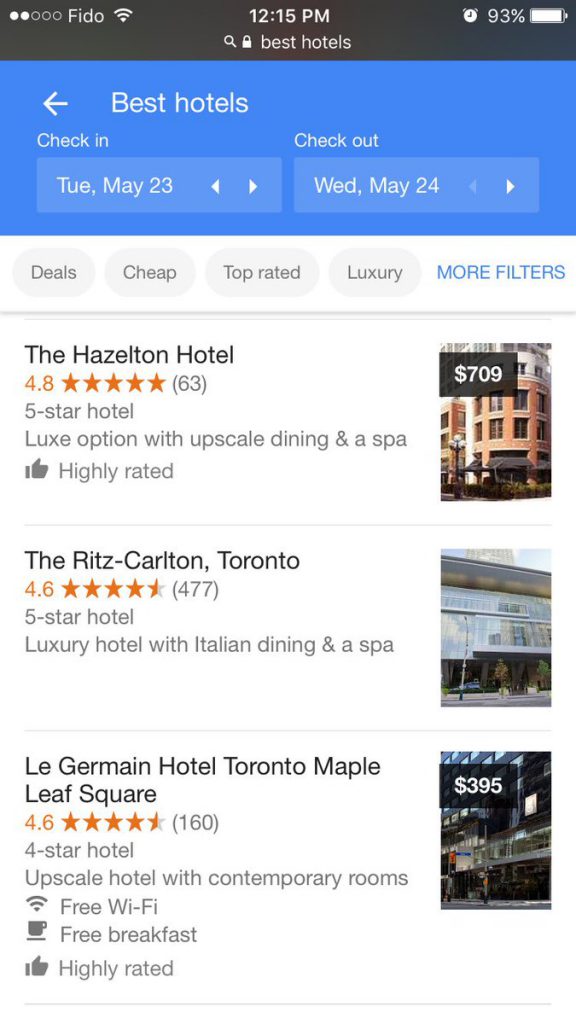This detailed caption describes a travel booking application's user interface:

The interface of a travel booking app is displayed against a white background. The interface shows the current time as 12:15 p.m., battery percentage at 93%, and the network carrier as FIDO. A small alarm clock icon is present on the screen. At the top section, a blue background strip displays the label "Best Hotels" with an arrow pointing to the left. Below this, the user can find check-in and checkout information: "Check-in: TUE, May 23rd" and "Checkout: Wed, May 24th."

Additionally, the interface features filters for narrowing down hotel options: "Deals," "Cheap," "Top-rated," and "Luxury," along with a "More Filters" button highlighted in blue. 

Three hotel options are displayed on the screen:

1. **Hazeltown Hotel**: 
   - Rating: 4.8 stars 
   - Reviews: 63 
   - Category: Five-star hotel

2. **The Ritz-Carlton, Toronto**: 
   - Rating: 4.6 stars 
   - Reviews: 477 
   - Category: Five-star hotel 
   - Price: $709 

3. **Le Germain Hotel, Toronto, Maple Leaf Square**

This comprehensive layout highlights user options and pertinent information for booking a stay at high-end hotels.